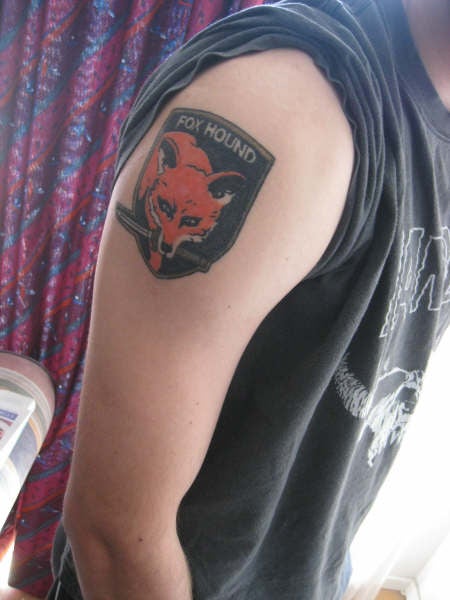The image features a close-up view of a man from the neck down to his waist, predominantly focusing on his right upper arm where he sports a detailed tattoo. The man is wearing a black t-shirt, with the sleeve rolled up to reveal the tattoo. The tattoo, resembling a shield crest, depicts a red or orange fox with a knife in its mouth, and above the fox, the word "FOXHOUND" is inscribed in capital letters. The man is standing sideways to the camera, obscuring his face but providing a full view of the tattoo. The background consists of a red and blue curtain that occupies part of the left-hand side of the image, while the rest remains dominated by the man and his tattoo. The overall setting gives the impression that the photo was taken indoors, possibly in a house.